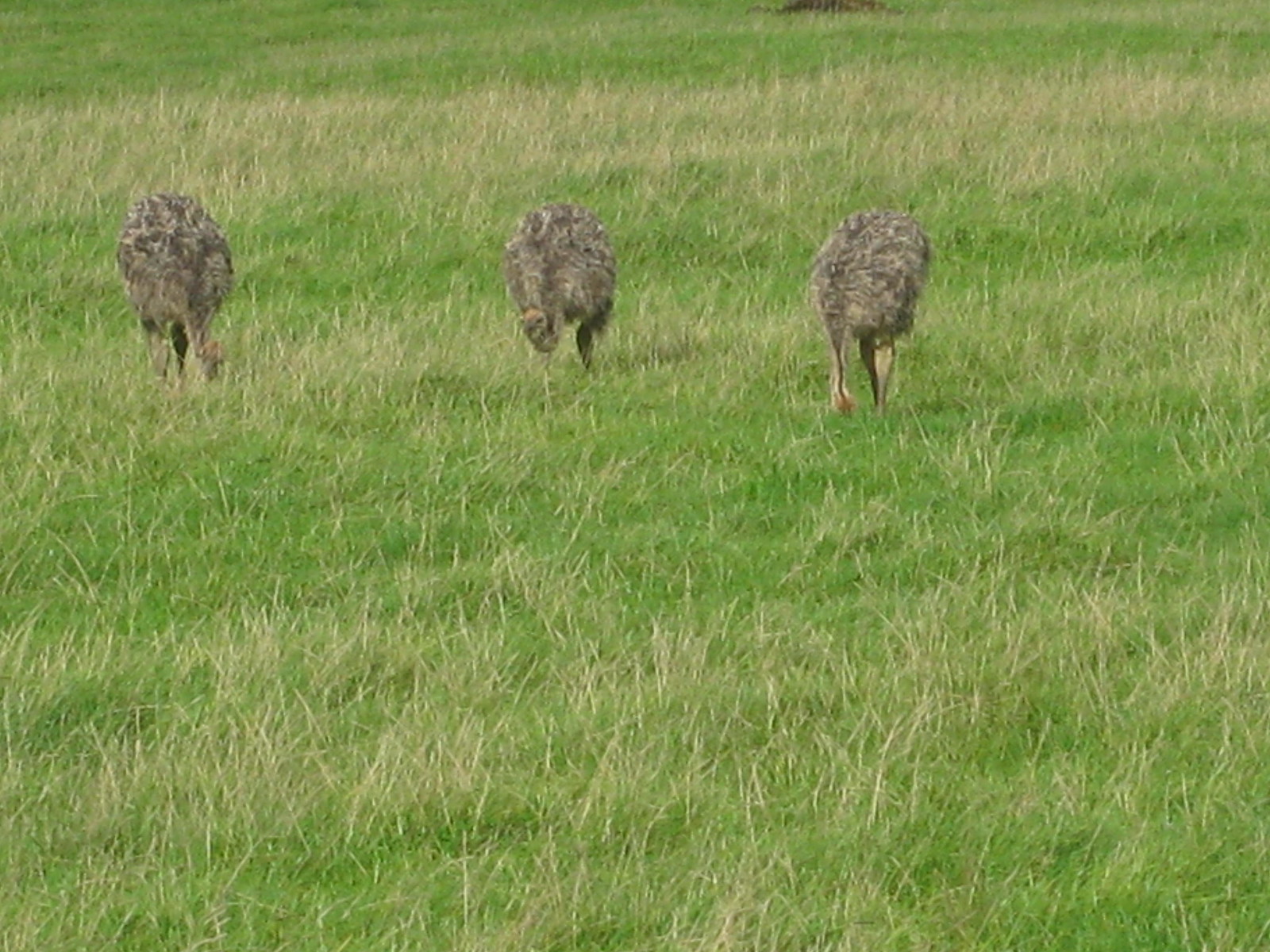In a sunlit grassy field, three large birds, resembling either emus or immature ostriches, are scattered near the top of the low-quality, slightly out-of-focus photograph. The field is a mix of tall, dried brown grasses and lush, bright green patches. The birds' plumage appears in shades of grayish-beige with lighter highlights, while their long legs look powerful and gray. All three birds have their heads down as if pecking or searching for food, except the middle one, which briefly lifts its nearly bare, fuzzy neck. The bright sunny day casts light across the scene, adding to the natural ambiance of this outdoor wildlife snapshot.